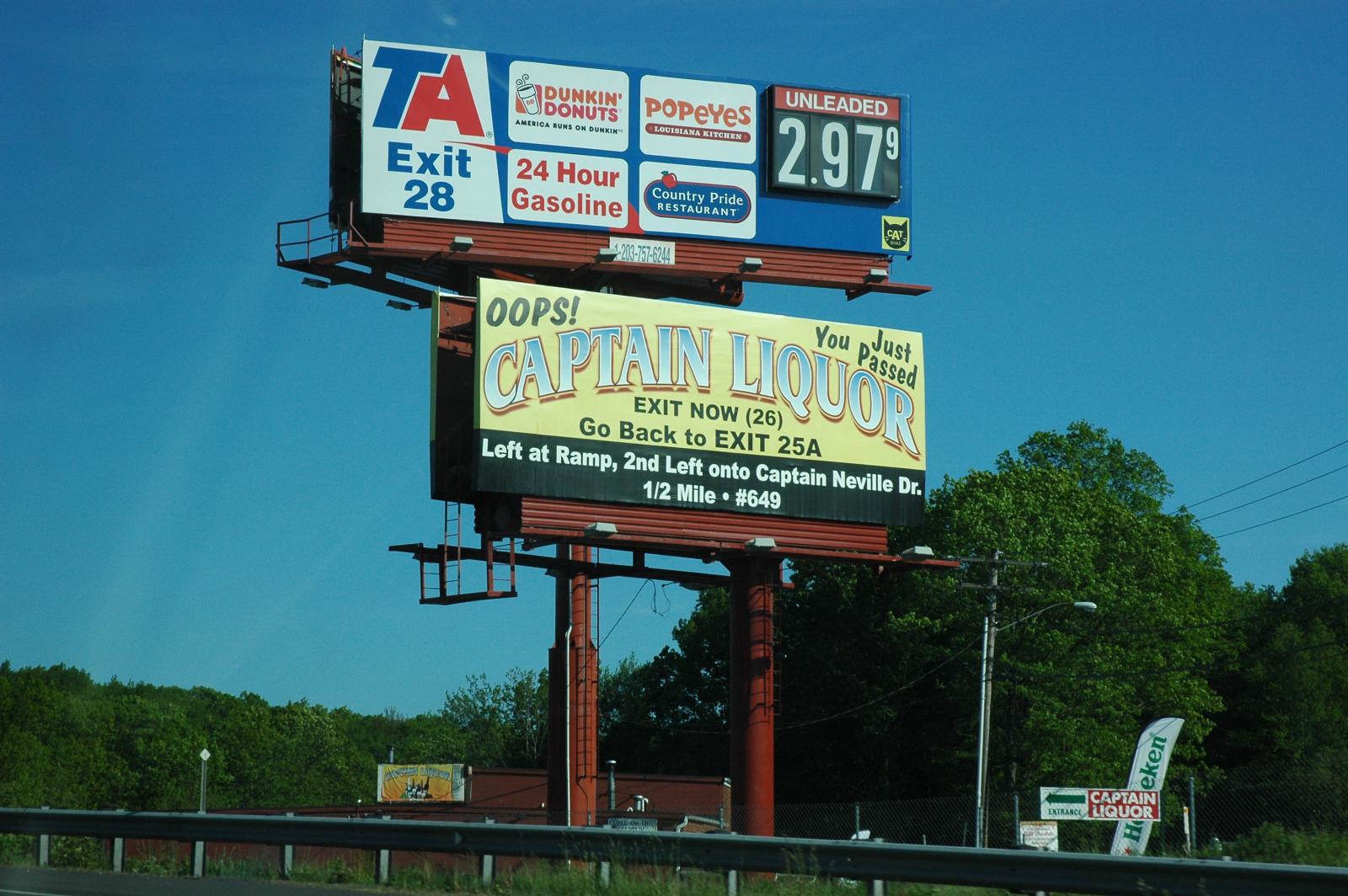The image captures two large billboards set outdoors on red-painted metal scaffold posts, standing approximately 30 feet high. Positioned along a roadway, identified by a visible guardrail, the scene is framed by a clear, blue daytime sky and encircled by numerous trees.

The top billboard features a blue background with several white rectangles displaying various ads: on the left, "TA Exit 28" in blue and red text; to its right, "Dunkin' Donuts" in orange and pink; next to it, "Popeyes" in orange; below, "24-Hour Gasoline" in red text; and finally, "Country Pride Restaurant" with a blue logo. To the top right, there is an adjustable sign reading “Unleaded 295.9.”

The lower billboard sports a yellow background with extensive text: "Oops, you just passed Captain Liquor, exit now 26, go back to exit 25A, left at ramp, second left onto Captain Neville Drive, half a mile," and a white number "649."

The overall composition vividly depicts a typical roadside advertising cluster, enhancing the realism with the inclusion of common details such as brand names, exit instructions, and a roadside setting.